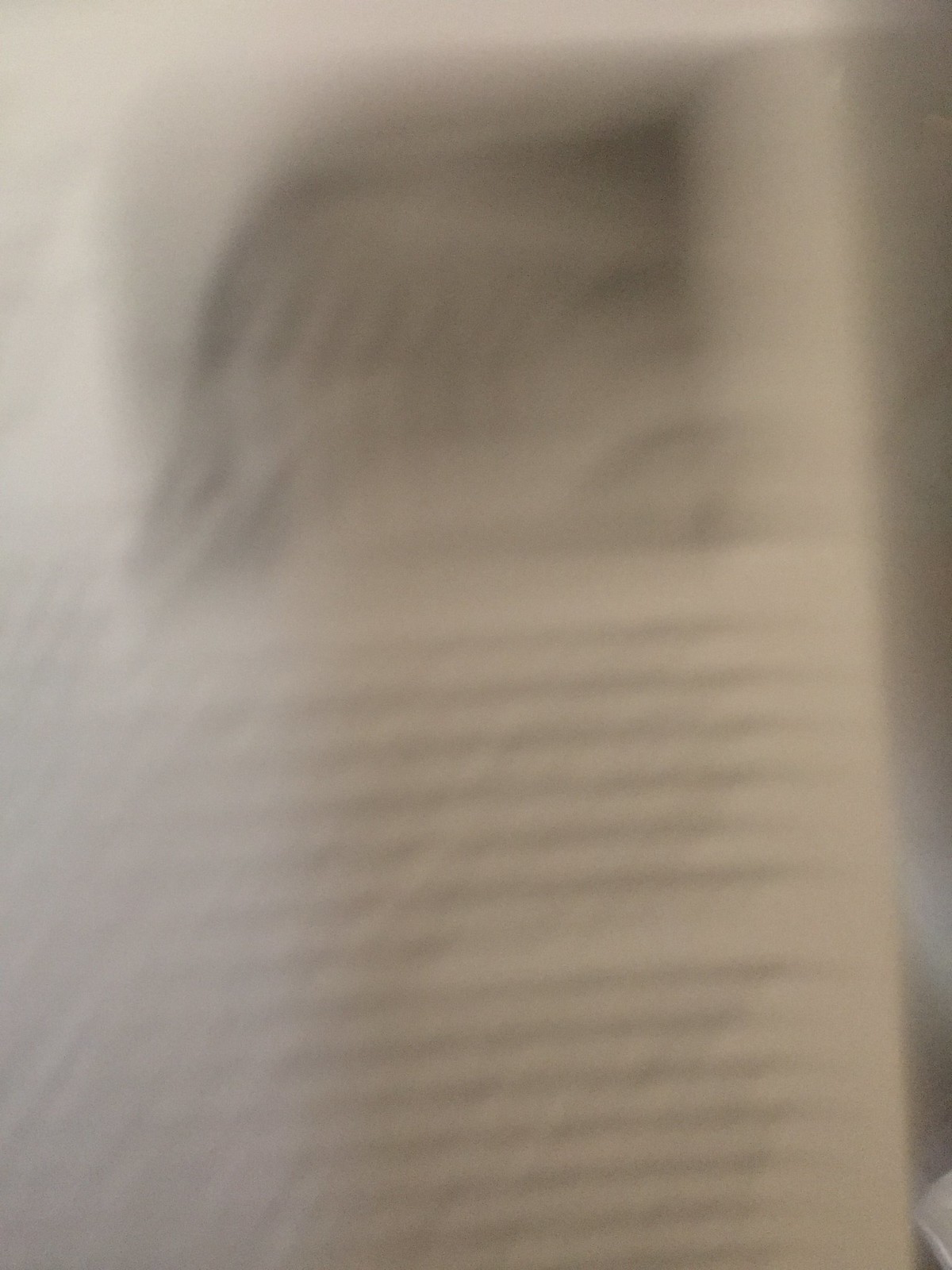A grainy image of an open book page is set against a neutral gray background. The top of the page features a prominent, slightly bent square image with a dark coloration, suggesting the presence of multiple, somewhat indistinct group photos. The lower part of the page displays a lighter tone, possibly due to the reflection of light, which also highlights the left edge of the page. The text on the page is printed in a darker ink, offering a stark contrast to the lighter areas around it, creating a varied texture and tone throughout the image.